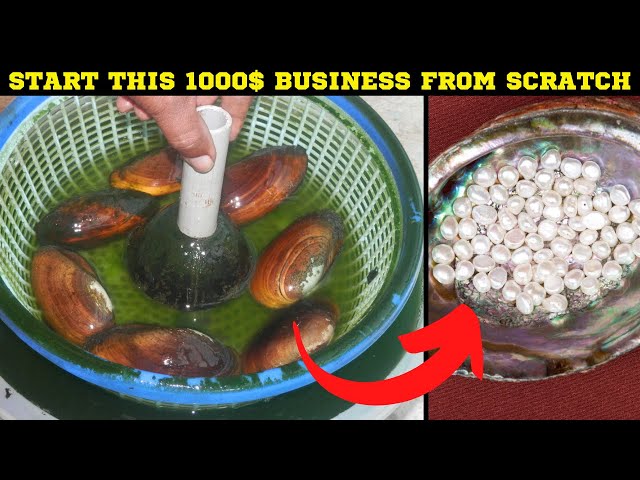The advertisement, set against a black background, prominently features the bold yellow text at the top: "Start this $1,000 business from scratch." Below the text, the ad is divided into two photographs. On the left, a person's hand partially visible, holding a white tube above a blue strainer filled with water and approximately seven brown-hued clams or oysters submerged in green liquid. The background of this side also includes white netting. An arrow from the strainer points to the image on the right, which displays a red tray filled with an assortment of glistening white pearls, suggesting the transformation from unopened clams to valuable pearls. The entire composition is bordered by black bars at the top and bottom, enhancing the contrast and focus on the depicted process and its lucrative potential.